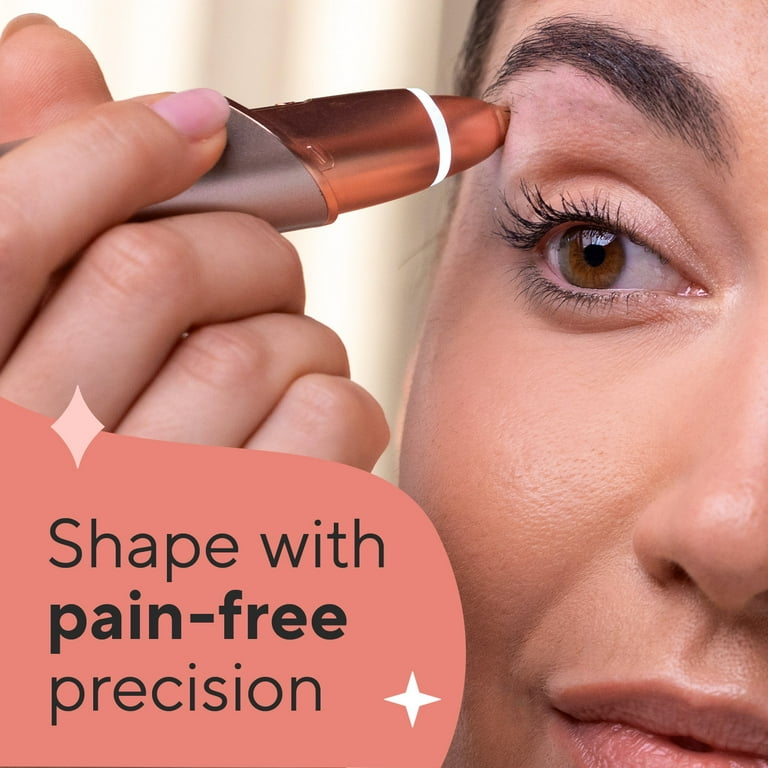The image depicts a close-up view of a Caucasian woman with dark hair and brown eyes, meticulously shaping her eyebrows using a device that closely resembles a thick tube of lipstick. She is seen facing a mirror, running the brow shaper across the lower portion of her eyebrow with her right hand, while her pink-painted fingernails add a neat touch to her appearance. The device, gray with a golden or almost pinkish sheen, emphasizes precision and pain-free application. This makeup advertisement prominently features an overlay with a desaturated orange background and bold black text stating "Shape with Pain-Free Precision," where "pain-free" is highlighted for emphasis. A diamond shape embellishes the word "shape," and a four-point white star appears to the right of "precision," accentuating the advertisement's promises. The woman's serene expression and focused eyes illustrate the product's ease of use and effectiveness in maintaining her eyebrows.